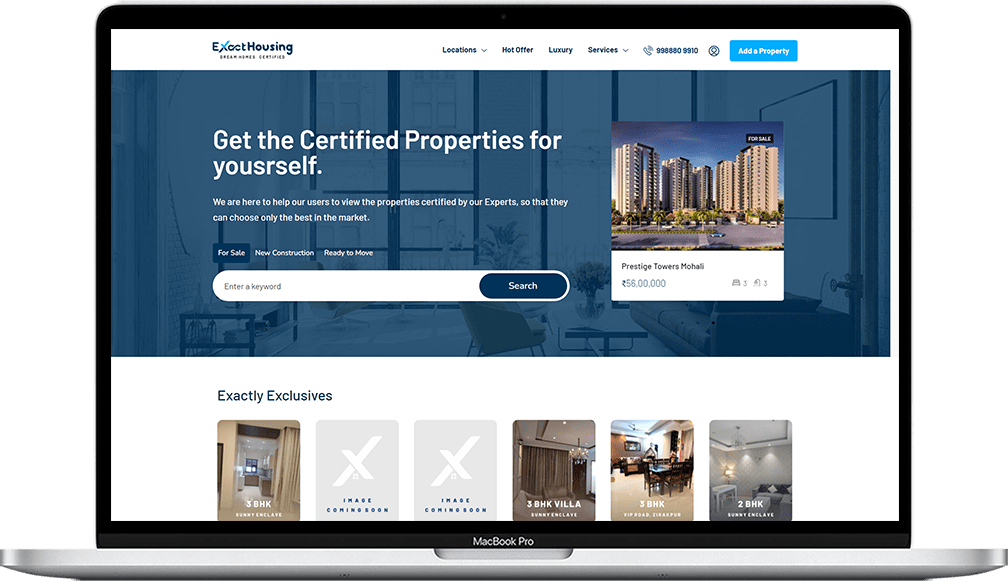A close-up photograph showcases the Exact Housing website displayed on a laptop, emphasizing the digital platform's user interface and design. The website features a distinct logo, "Exact Housing," with the word "Exact" highlighted by a green 'X' and the rest of the text in blue, set against a blue background with white font. The navigation bar, styled in white, guides users through various aspects of the site.

The primary focal point of the website is its offering of certified, exclusive properties that are available for purchase or rental. A prominent headline reads, "Get the certified properties for yourself," enticing visitors to explore the high-quality listings. The website provides detailed images of various apartment buildings, complexes, and condominiums, each accompanied by information about unique offers and contact options. Users are also given the opportunity to register their property or browse available listings. The central purpose of Exact Housing is to facilitate the acquisition of exclusive rental properties that might typically be inaccessible in the general market.